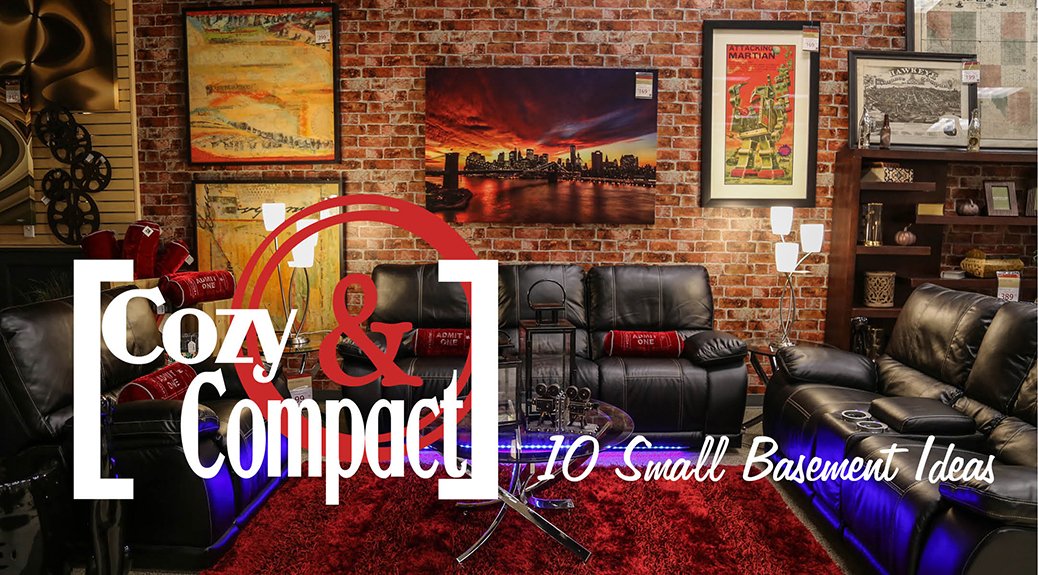The photograph appears to be a magazine article image titled "Cozy and Compact, Ten Small Basement Ideas." The setting is a stylish and cozy living room, possibly located in a basement. The room features a prominent brick façade wall adorned with four large pieces of framed canvas art, including a striking city skyline centerpiece. Three black leather couches are arranged in a rectangular seating configuration: one against the brick wall, and two facing each other on the left and right. A vibrant red deep-pile rug anchors the seating area, complemented by a central coffee table with a lantern. A bookcase filled with objects, including film reels, adds a touch of sophistication on the right side.